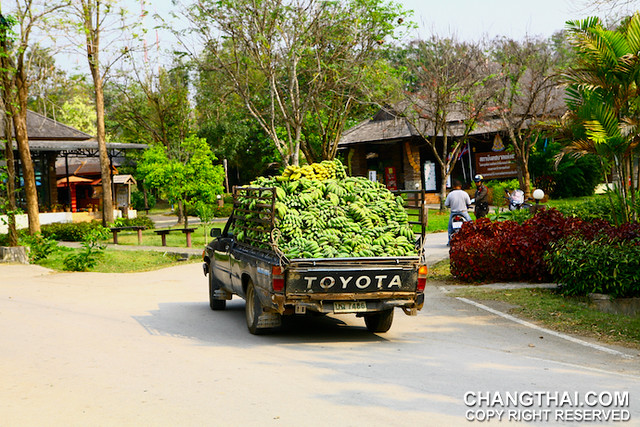In this detailed photograph, an old, rusty brown Toyota pickup truck loaded with a large quantity of green bananas is the focal point. The vehicle, with distinct white "TOYOTA" text on its rear, is moving along a driveway towards a cluster of low-rise buildings that seem to be part of a market or farmhouse setting, possibly in Asia. Surrounding the truck are lush green bushes, with a noteworthy deeper red-colored bush on the right side that stands out among the greenery. In the background, people can be seen standing, suggesting a bustling, communal atmosphere. Additionally, a man on a motorcycle or moped wearing white clothes is visible ahead of the truck, with another person in brown clothing nearby. A path leads to a building on the left, adding to the intricate setting of the scene. At the bottom right corner of the image, the website "shangthai.com" is prominently displayed in white bold letters, accompanied by a "copyright reserved" notice.